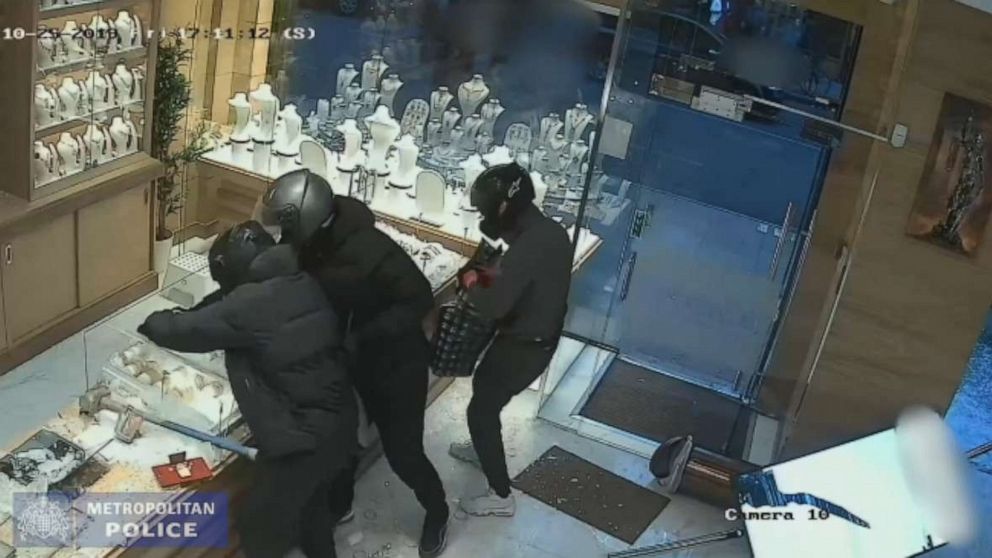The image depicts a dramatic scene captured by a security camera inside a jewelry store. The store's interior features glass cases filled with various pieces of jewelry, including mannequins adorned with necklaces. The focal point of the image is three individuals, each dressed in black and wearing black or gray motorcycle helmets, seemingly engaged in a robbery. Two of the thieves are clad in black and gray winter coats, adding to their concealed appearances. They appear to be breaking into the glass cases and taking jewelry, with a knocked-down trash can and shards of broken glass scattered on the floor indicating the violence of the scene. Notably, the bottom of the image is marked with the text "Camera 10" and "Metropolitan Police," suggesting it is a still from a security feed. On the right side of the image, an open doorway is visible, indicating a possible point of entry or escape.